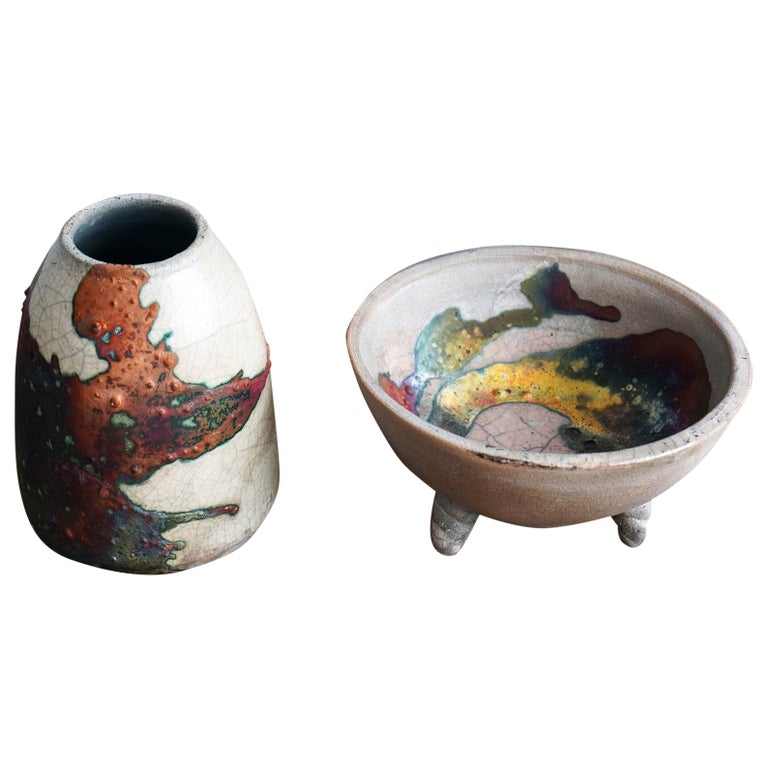This horizontal image features two pieces of striking ceramic pottery. On the left side, there's an elegant vase with a narrow neck that gradually widens into a broader body. The vase is predominantly white with a cracked and glazed texture, adorned by an abstract design with splotches of color. The design starts at the top with shades of orangey hues, blending into darker tones towards the bottom. These colors sporadically include hints of blue and red, enhancing its artistic appeal with an amorphous quality that’s intriguing yet undefined.

On the right, a distinctive bowl with three stubby legs is visible, slightly tipped to reveal its interior. This bowl, also crafted from cream-colored ceramic, features an inner surface decorated with vibrant splashes of yellow, black, blue, and red. The interior shares the same cracked and glazed appearance as the vase, tying the two pieces together thematically. The bowl's design is reminiscent of a detailed map, adding a layer of complexity to its aesthetic. Both pieces are hand-crafted, showcasing skilled artistry and a shared color palette that includes browns and blues, emphasizing their attractive and complementary styles.